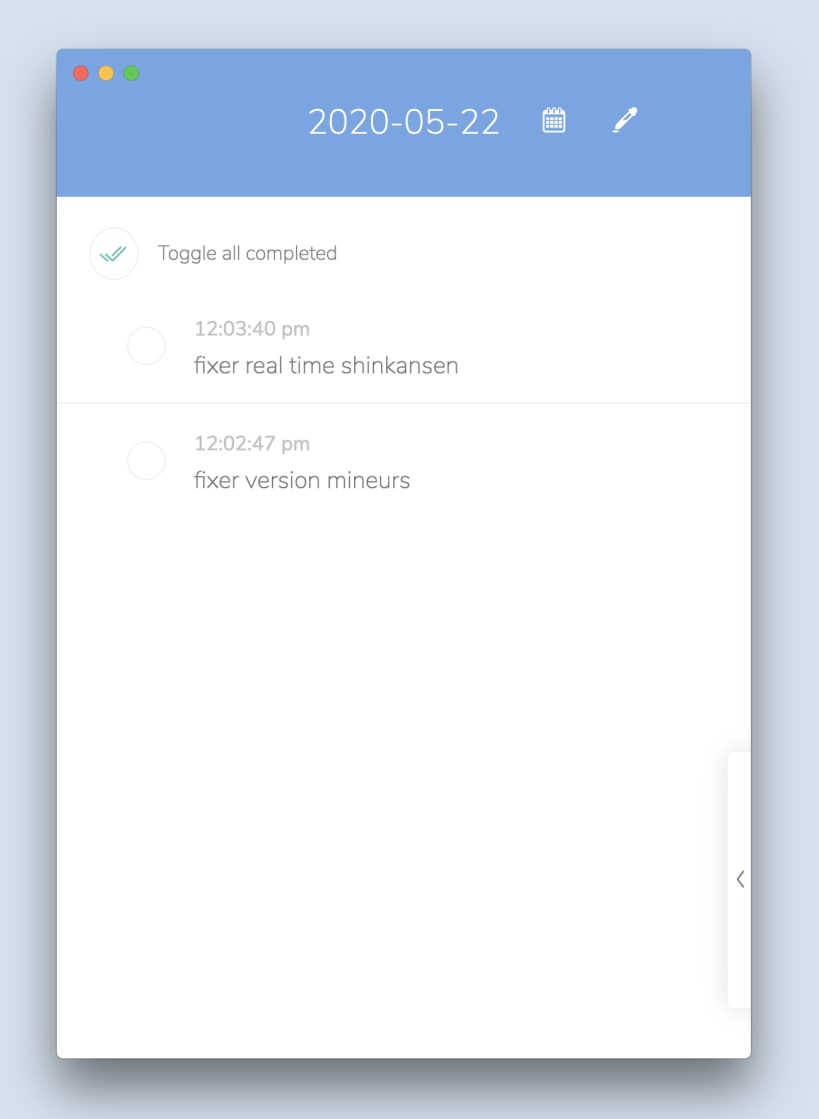An image of a simple website is displayed against a light blue background. The website features a darker blue header at the top. In the upper left-hand corner, there are three dots, colored red, gold, and green, arranged horizontally. Below these, the date "2020-05-22" is prominently displayed next to small icons of a calendar and a pen.

The main section of the website is white, starting with a feature labeled "Toggle all completed." To the left of this text is an image of a circle containing two green check marks. 

Further down the page, in black text, the timestamp "12:03:40 p.m." is followed by the label "Fixer real-time Shinkansen," next to a circle that is empty. A light gray horizontal line separates this entry from the next.

Below the line, the text "12:02:47 p.m." is displayed, followed by the label "Fixer version manures," also with an adjacent empty circle.

On the bottom right side of the website, there is an inset that resembles a browser window emerging from the side. This inset features a gray arrow icon pointing outward.